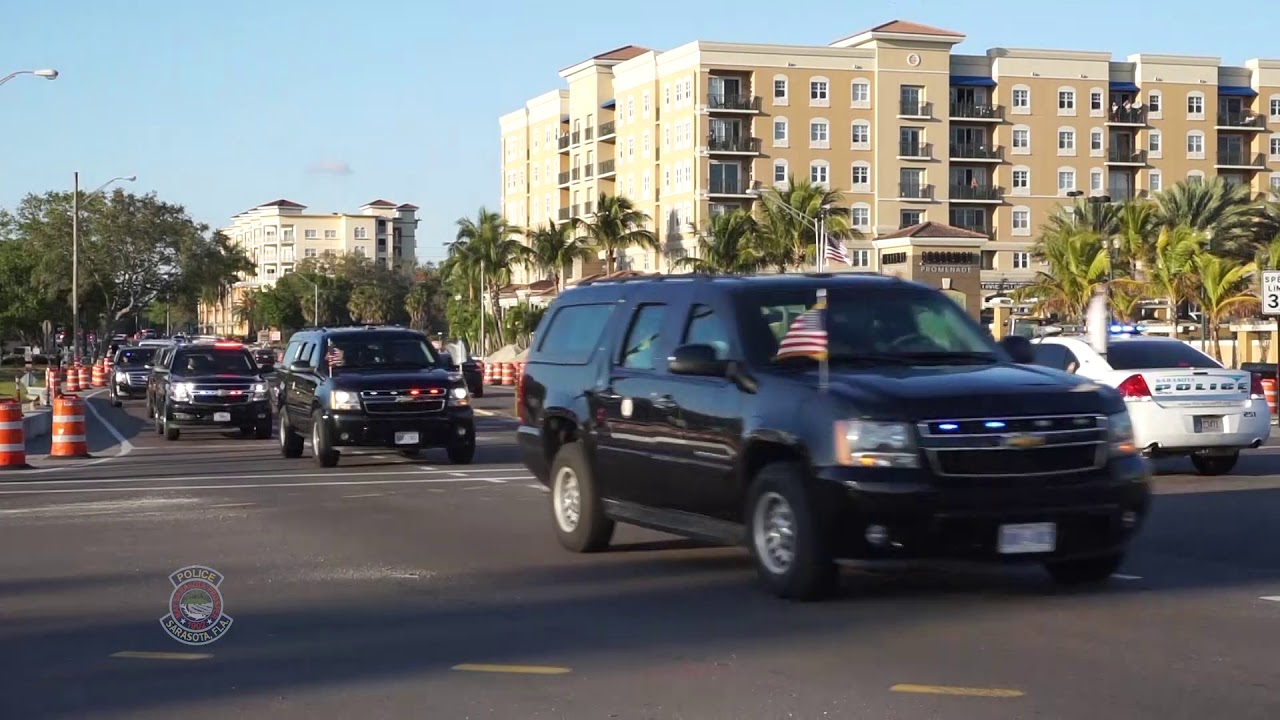The photograph captures a presidential or vice-presidential motorcade navigating through a sunny, tropical area, likely Sarasota, Florida, as indicated by a watermark on the image. The motorcade consists of five shiny black SUVs, specifically black Suburbans, each adorned with American flags on the right front hood. One of the SUVs features a light bar on top. There are orange traffic cones blocking off traffic to the left side of the street, where a police car ensures the procession's smooth progression. The background showcases a series of large, high-rise apartment or condo buildings, ranging between six and eight stories, in a sandy beige color with terracotta roofs. Numerous palm trees dot the scene, adding to the tropical ambiance under a clear, blue sky with warm sunlight illuminating the buildings.